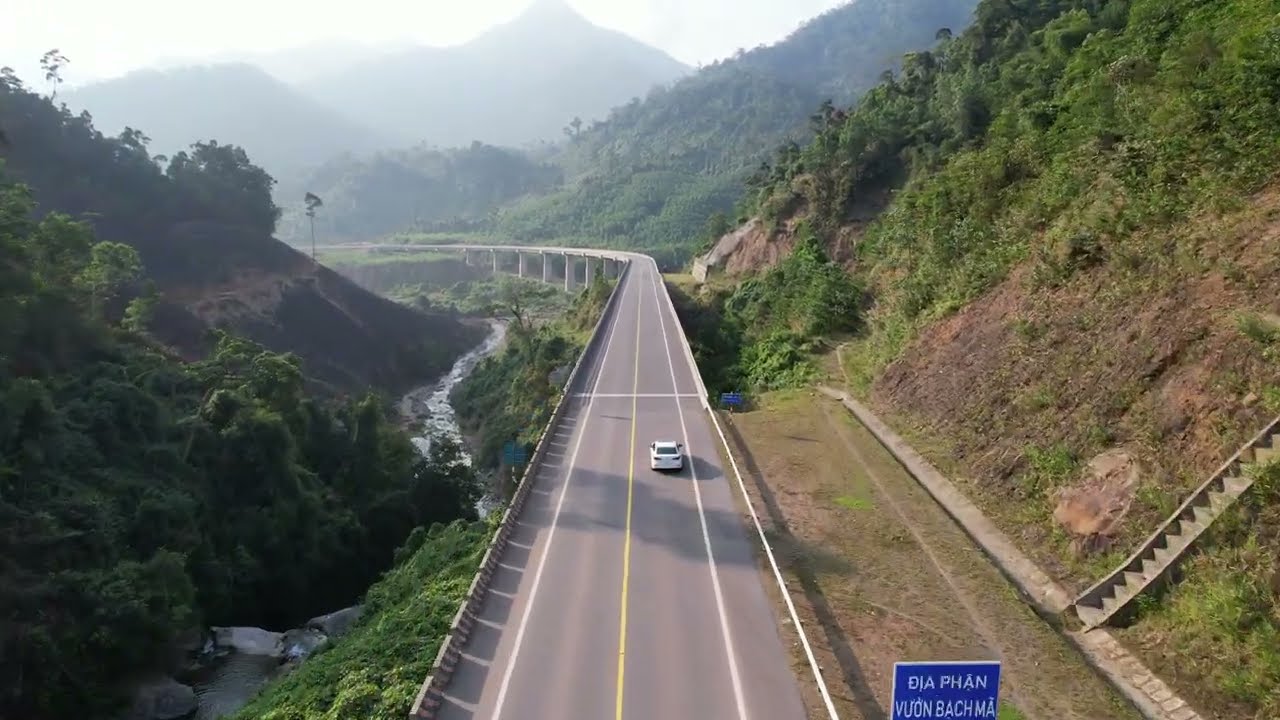This photograph, taken from a point of elevation, captures a two-lane roadway extending from the foreground to the distant center of the image before curving off to the left. The road, featuring a single yellow line in the center and white lines on either side, is composed of gray-black concrete. It accommodates a white car traveling along its stretch. The roadway is a bridge supported by large gray cement pillars, crossing over a meandering stream on the left side. This stream marks the beginning of verdant hills densely covered with green foliage, including bushes and trees, which continue into the distance. On the lower right-hand side, a stone staircase ascends the hillside. A sign reading "Dia Phan Yuen Bachma" is visible along the road, adding a cultural touch to the scenic and intricate landscape. The sky above is slightly blurred, giving a hazy backdrop to the majestic, mountainous setting.